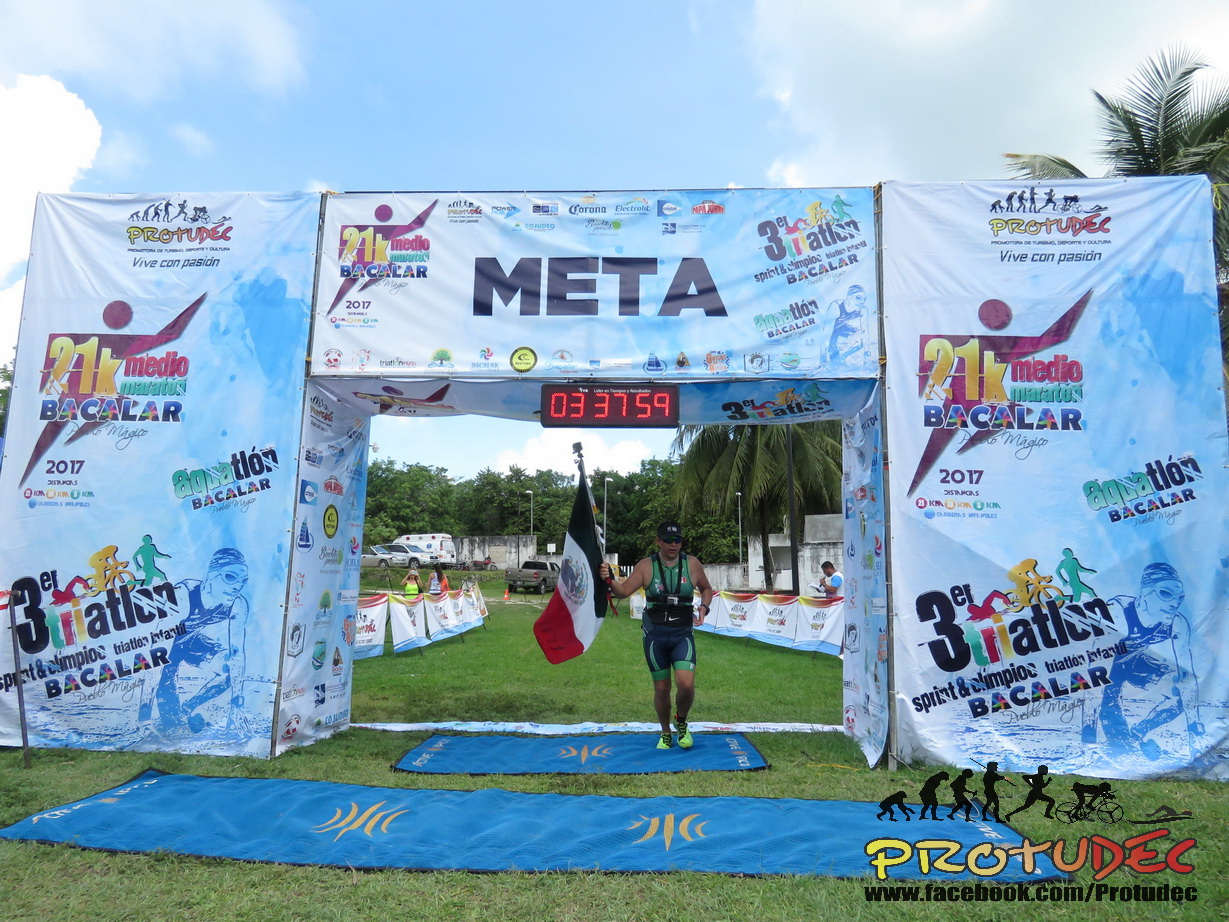The image captures a dynamic scene at the finish line of a race, featuring a fit, tanned runner with a Mexican flag in one hand. He is dressed in a green tank top, dark blue shorts, light green shoes, and a black hat. The setting is dominated by a rectangular arch adorned with various event logos and text, including prominent displays for "3ER Triathlon Sprint and Olympian Barcalar" and "21K METEO Barcalar," accompanied by stick-figure icons and color schemes of green, red, and blue on a sky-like background of white and shades of blue. The central sign prominently reads "META" with a time of "03:37:59" displayed beneath it. 

In the bottom right corner, a logo for PROTUDEC is visible with an evolution chart illustrating a monkey transforming into a sprinting man and finally into a cyclist, alongside the text "facebook.com/protudec." The foreground features dark blue carpeting with golden vertical lines, extending under the runner. Background elements include some fencing, trees, parked cars, and a partly cloudy sky with a slightly visible palm tree peeking from the top right. With detailed event signage and a vibrant scene, the photograph captures the triumphant moment as the runner crosses the finish line.